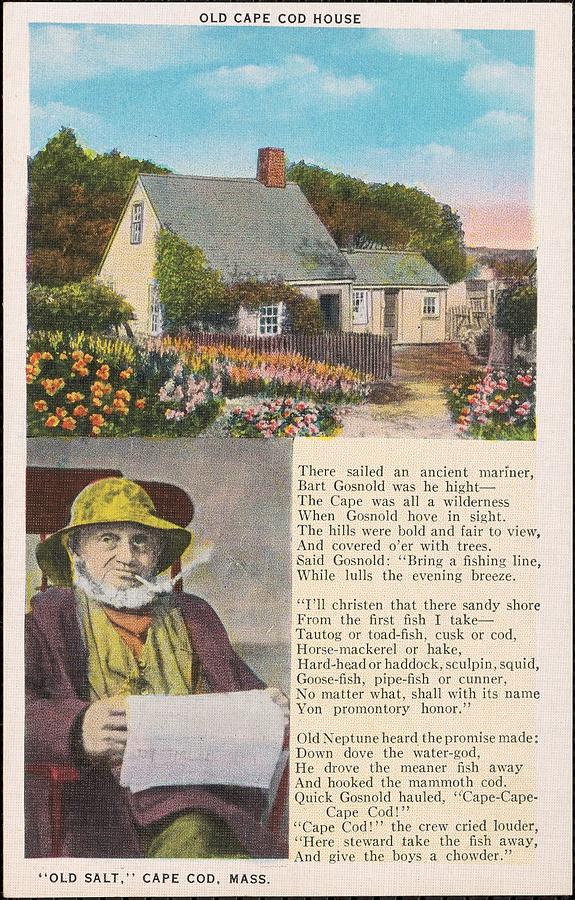This image appears to be a vintage postcard or a page from an old picture book or magazine titled "Old Cape Cod House." The top section features a painting of a quaint, two-story Cape Cod house, adorned with a lush flower garden in the foreground and framed by trees. The sky above is a picturesque blue with a few scattered white clouds, adding to the serene ambiance. 

In the bottom left of the image, there is another painting depicting an elderly seafaring man dressed in a yellow slicker and hat, with a bushy chin-strap beard and no mustache, smoking a cigarette. The man appears to be gazing directly at the viewer, holding a newspaper that seems to be falling from his hand. This section of the image is labeled "Old Salt Cape Cod, Massachusetts" and includes a poem written in older English, adding a historical touch to the scene.

A descriptive caption accompanies the image, providing further context and emphasizing the charm and historical essence of both the house and the seafaring figure.